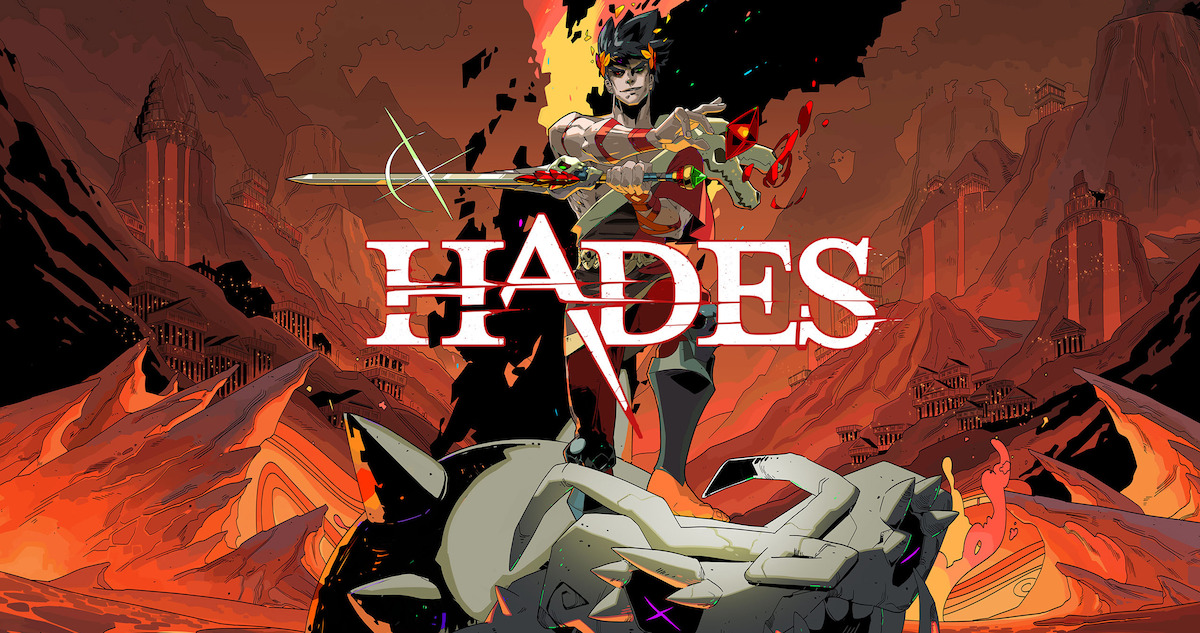This digital artwork, reminiscent of a comic book's frontispiece or a section title page, prominently features the word "HADES" in sharp, white, all-caps lettering centered across the scene. Dominating the image is a male warrior with black spiky hair, seemingly ablaze with fiery energy and adorned with orange leaves beside his head. His eyes are strikingly mismatched—one green and one red. The warrior stands upright, his right arm extended in front of him, wielding a sword that points horizontally to the left. His left foot is propped up on what appears to be a slain horse, though it's difficult to discern clearly. This figure wears shin armor, and at his side, a yellow diamond core is visible, adding to his formidable appearance. The background is a chaotic blend of jagged rocks and towering mountains shrouded in smoke, with small buildings precariously perched on cliffs. The image is accented by intense orange flames at the bottom, enhancing the infernal visual theme of "Hades."